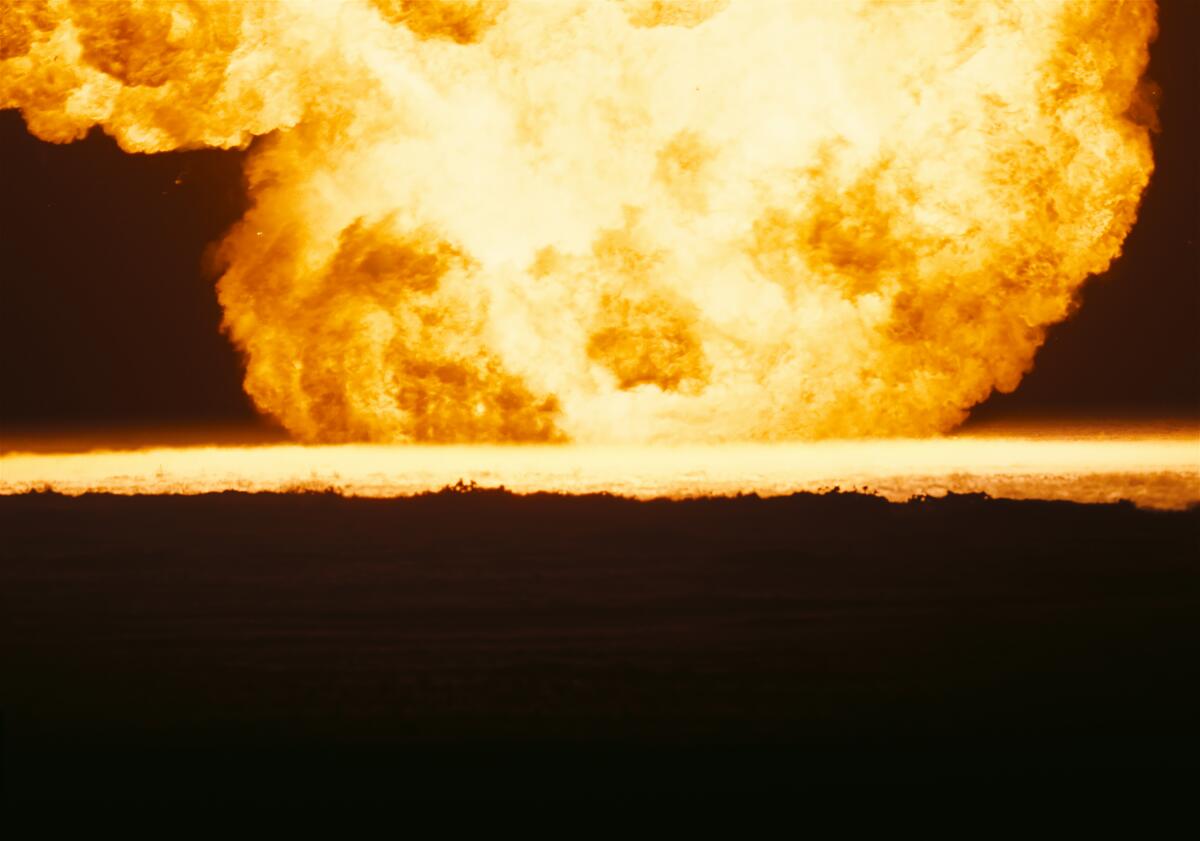The image captures a dramatic and intense explosion, suggesting the detonation of a massive weapon, such as a nuclear or hydrogen bomb, during nighttime. The bottom half of the image is engulfed in complete darkness and shadow, lending a stark contrast to the fiery explosion above. In the background, a horizon line of blazing fire stretches across the top center of the image, radiating with vivid hues of orange, red, yellow, and white. These colors merge to create a spectacle reminiscent of a fiery planet or a surreal scene from another world. The explosion dominates the upper half, resembling a gigantic mushroom cloud with a smoking fireball at its core. The unnaturally black sky further accentuates the luminous, fiery display, creating a mesmerizing yet alarming visual of sheer destruction and raw power.